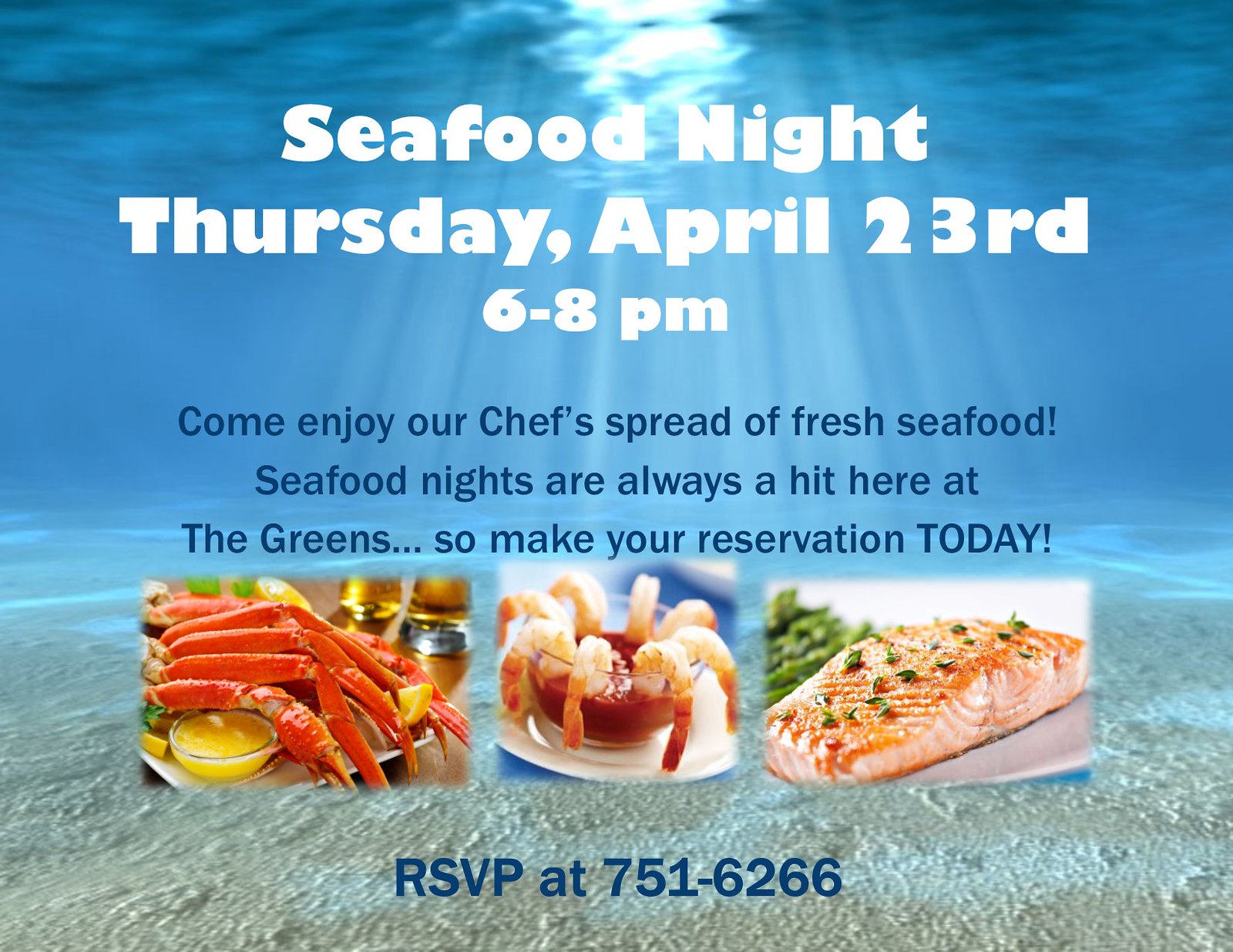The advertisement is a vibrant and engaging promotion for "Seafood Night" taking place on Thursday, April 23rd, from 6 to 8 p.m. at The Greens. Set against a striking background of an underwater scene, the image beautifully captures the ocean floor bathed in sunlight filtering through the water. The main text, displayed in white, prominently announces the event details, with accompanying blue text inviting patrons to "Come enjoy our chef's spread of fresh seafood. Seafood nights are always a hit here at The Greens, so make your reservation today." For reservations, the contact number 751-6266 is provided. The ad includes three appetizing images of the featured seafood dishes: vibrant reddish-orange king crab legs served with yellow melted butter, a shrimp cocktail dish, and a beautifully garnished plate of salmon.